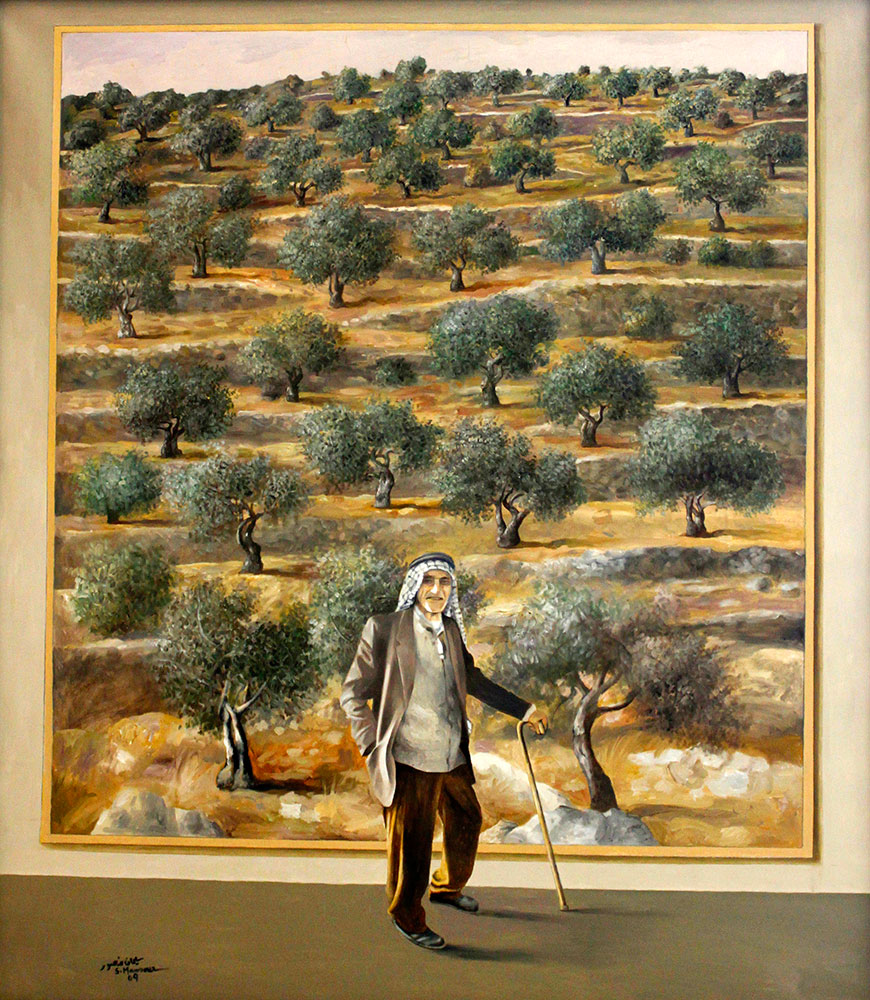The painting depicts an elderly Middle Eastern man wearing a traditional white and black headdress secured with a black headband. He has a light, white beard and is dressed in a brown suit jacket over a gray-ish sweater, with a white T-shirt peeking out underneath. His dark tan dress pants complement his black dress shoes. The man's left hand grips a walking cane that touches the ground, while his right hand rests in his suit pocket. He stands facing the viewer, positioned in front of a colossal painting that towers at least three times his height, dominating the background. This secondary painting portrays a vast environmental scene featuring rocky hills or dunes, dotted with various short trees and a few scattered rocks, under a glimpse of sky. The sense that this artwork might be part of a museum collection is heightened by the grand scale of the background painting, creating a visual effect of a painting within a painting. The floor beneath the man is a dark tan or tannish green hue, and though slightly obscured, the artist's signature appears in the lower left corner.